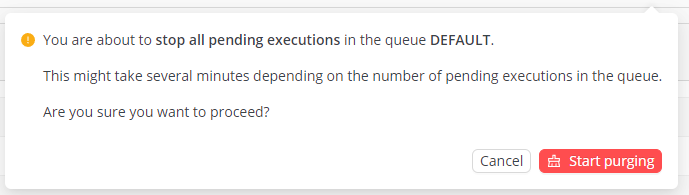The image displays a pop-up notification box on a webpage with a light gray background featuring horizontal lines. The central element is a white rectangular box, resembling a pop-up window. At the top of this pop-up, there is an orange circular icon with a vertical line through it. Beneath this icon, the text prominently reads, "You are about to stop all pending executions," with the phrase "stop all pending executions" rendered in bold. Additionally, "IN THE QUEUE" follows this, with "QUEUE" in all caps and also bolded in black.

The message continues, stating, "This might take several minutes depending on the number of pending executions in the queue." Below this, the text asks, "Are you sure you want to proceed?"

In the lower right-hand corner of the pop-up, there are two buttons: a gray "Cancel" button on the left, which is white text on a gray background, and a red "Start Purging" button on the right, which features white text and an icon. The icon is box-like with a small protruding part in the middle, resembling a crown.